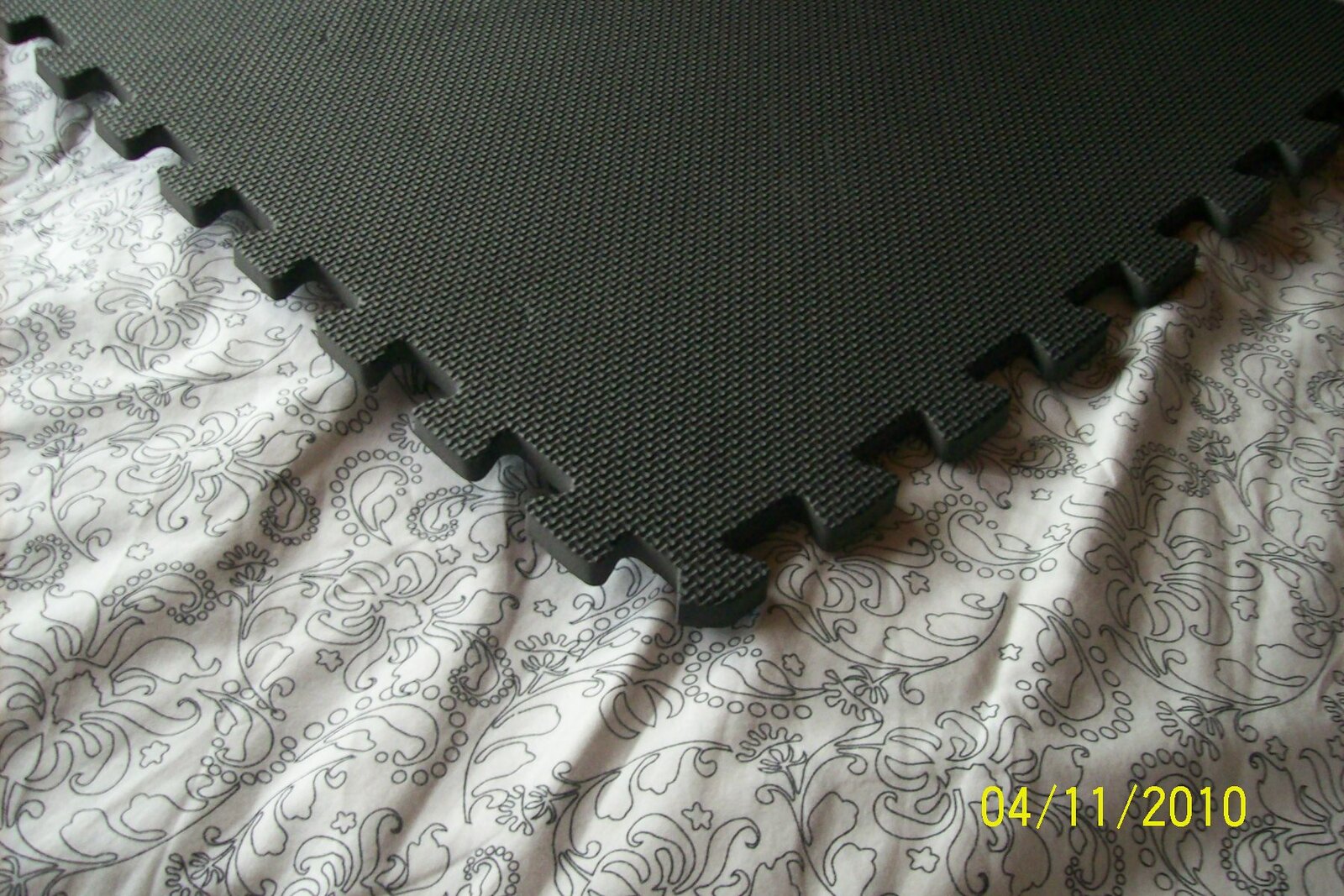The image is a color photograph capturing a scene with detailed elements. Positioned in the bottom right corner and slightly inset from the edges is a yellow date stamp reading "04.11.2010". Dominating the center of the image is a black corrugated foam tile, likely used as a playmat for children or as a temporary flooring surface in areas like drive-in car garages or for protecting floors under workout equipment. The foam tile features interlocking puzzle-like teeth, with 8 visible on the left side and 7 on the right. It has a waffle-like texture with small bumps across its surface.

The tile rests on a bedspread spread over a bed. The bedspread is a beige cream color adorned with a swirling pattern of flowers, stems, and leaves, creating a soft, delicate backdrop. The fabric is slightly ruffled, forming pleats that extend diagonally from the back right to the front of the frame. The combination of these elements, along with the date stamp, provides a vivid, descriptive scene captured in this photograph.